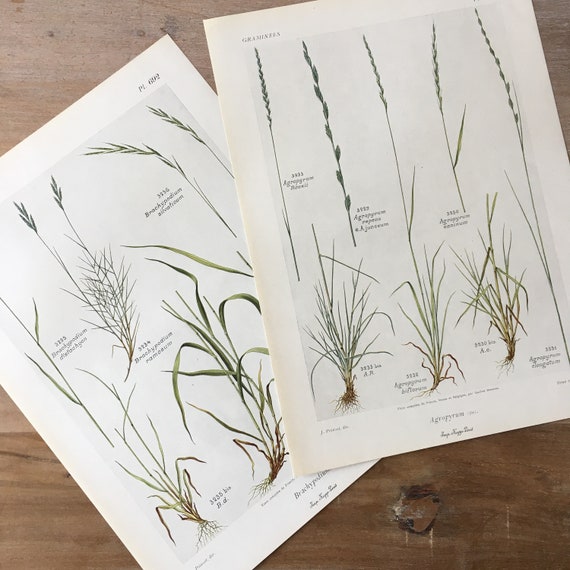A full-color, vertically rectangular photograph taken indoors using artificial light, captures two aged sheets of paper placed on a dark brown stained wooden table. The table, featuring visible wood grain and knots, notably one in the bottom right corner, adds a rustic backdrop to the scene. Each sheet of paper, approximately 8.5 by 11 inches, showcases artistically drawn wild plants, characterized by leaves at the bottom, long thin stalks, and seeds or flowers at the top, with green and brown hues dominating the illustrations. The sheets, slightly overlapping, have titles in the upper left, though the text is too small and blurry to read even when magnified. The lower sections of these drawings display the roots of the plants, extending into faintly detailed depictions of soil. Despite the small and partially cropped text sprinkled throughout, the image vividly details the delicate forms and structures of botanical specimens.